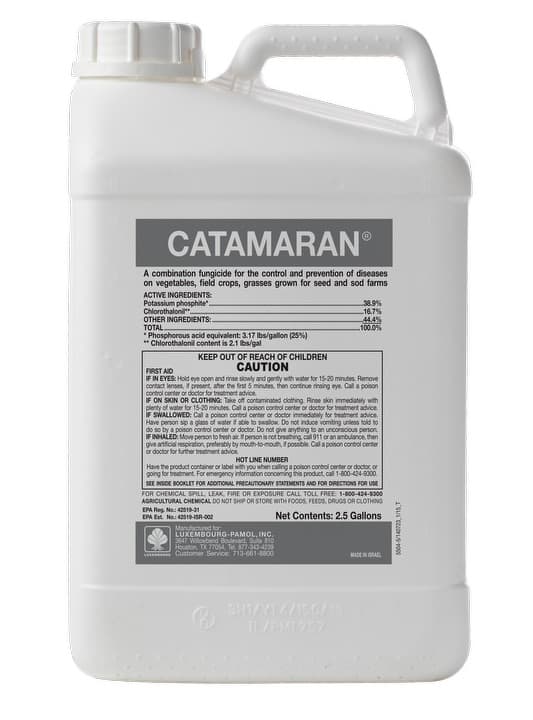This image features a large, white rectangular plastic jug labeled "Catamaran," a combination fungicide designed for the control and prevention of diseases on vegetables, field crops, grasses grown for seed, and sod farms. The jug has an integrated handle at the top, along with a white, round screw-on lid next to the handle. The front and center of the jug features a detailed label with a grey top and bottom section. The label highlights the active ingredients: Potassium phosphate (38.9%), Chlorophenol (16.7%), and other ingredients (44.4%), totaling 100%. Prominently displayed is a caution notice: "Keep out of reach of children." Additionally, there are first aid instructions including how to rinse eyes gently with water for 15-20 minutes if there is contact, and specific guidance for treatment if inhaled or swallowed. The product weighs the equivalent of 3.17 pounds per gallon, with a net content of 2.5 gallons. The jug is set against a bright white background, drawing attention to its utilitarian design and critical warnings.